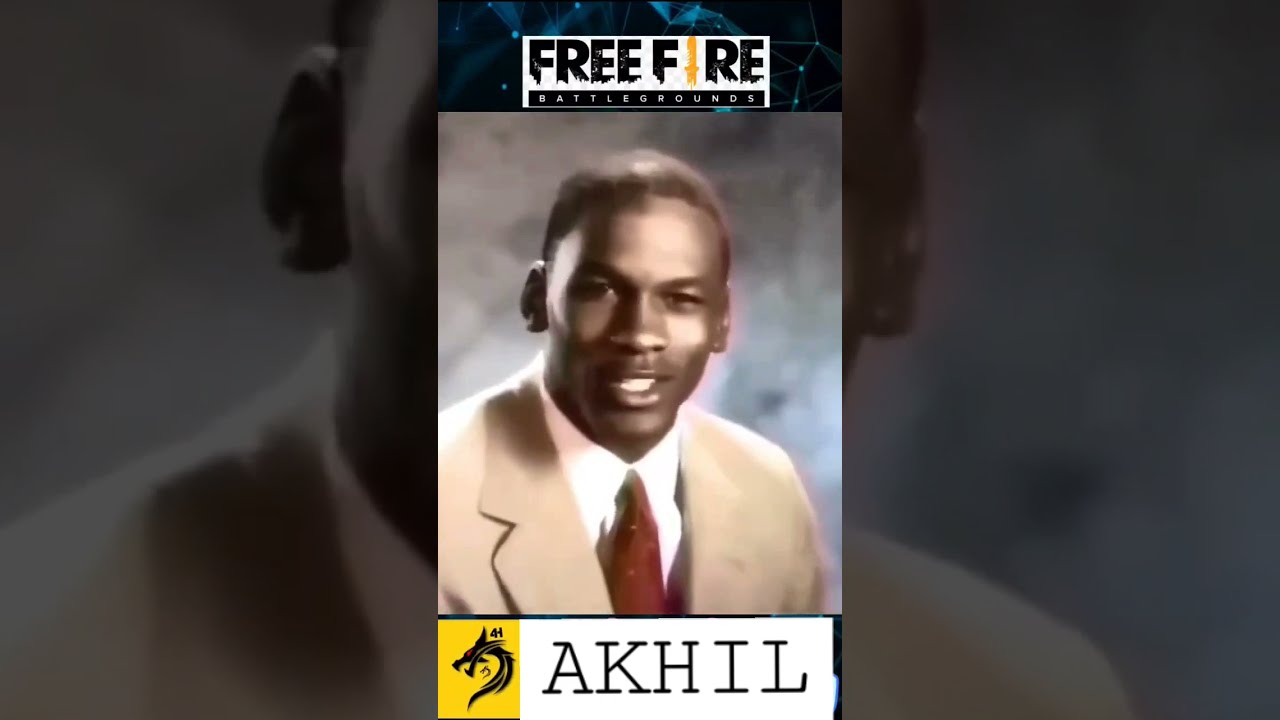The image features a younger Michael Jordan, captured in a headshot against a blotchy gray background. He is dressed in a beige or tan-colored suit, accompanied by a white button-down shirt and a burgundy tie. His expression is a half-smile with visible teeth, and he sports a short fade hairstyle. Above the picture is a banner reading "Free Fire," with the letter "I" depicted as a yellow sword. Below the image is a black banner that states "Battlegrounds" and features the name "Akhil" (A-K-H-I-L) along with a yellow dragon head symbol. Additionally, the background has elements resembling constellations, contributing a dark, cosmic feel.